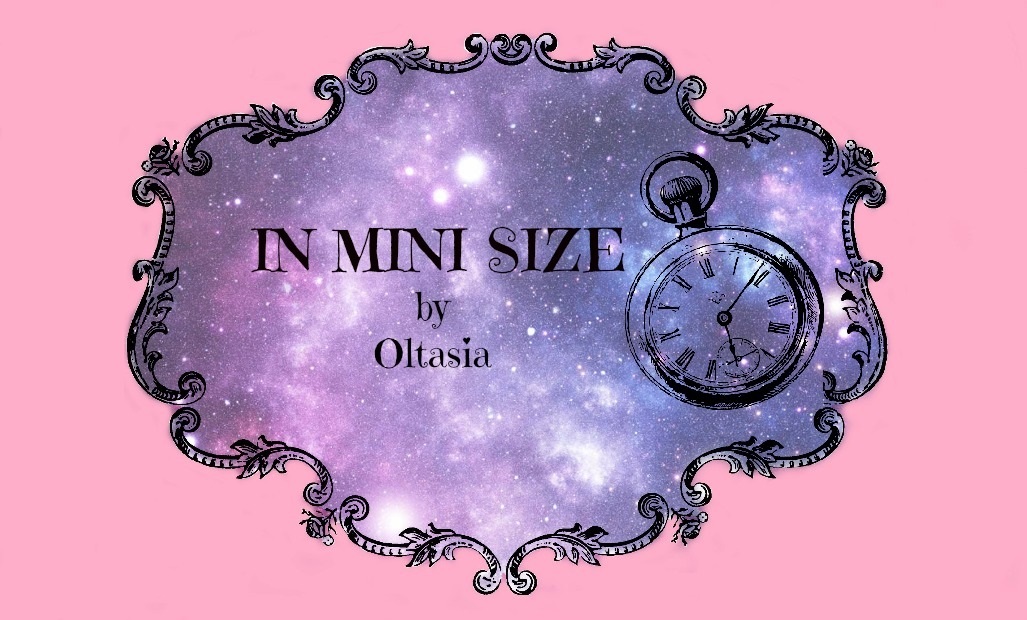The image presents a detailed, illustrated emblem set against a vivid pink background. The emblem, which features an intricate Victorian-style design with a black border, is a combination of celestial and temporal elements. At its center, the scene depicts a night sky teeming with hundreds of stars in various colors, predominantly in shades of purple, blue, and pink. Within this star-filled sky is an illustration of a pocket watch, complete with Roman numerals and watch hands, outlined in black and white, giving it a classic look. Above the watch is a stylized text, "in mini size by Oltasia," with "Oltasia" spelled out in all caps and a heart replacing the dot above the 'i'. The entire image exudes a sense of timeless elegance and cosmic wonder, encapsulated within the ornate, spiky-bordered emblem.